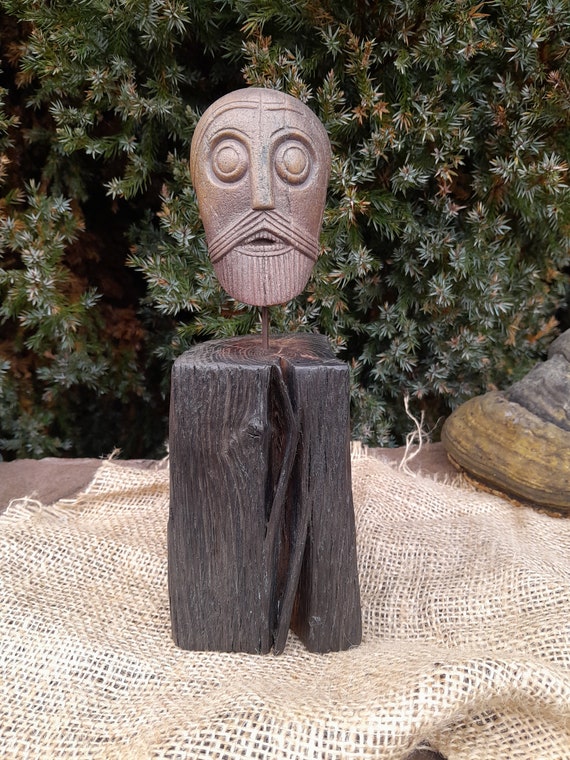This is a detailed photograph of a tribal-style mask, crafted from dark wood and mounted on a rustic base. The mask, around two feet tall, features an oval shape that broadens slightly at the top. It has intricately carved facial features, including wide, round eyes, a rectangular nose, a slightly open mouth, and a distinctive triangular mustache that slopes downward, connecting to a beard on the chin. The mask is affixed to a rusty metal stand that extends down into a dark brown, possibly stained, stump. The stump has a split and a spike protruding from its middle and rests on a piece of burlap spread out on a table. Behind the object, there is a dense thicket of pine and fir trees, with only the lower branches visible. This natural setting contrasts with the textured burlap and the dark tones of the mask and its base.